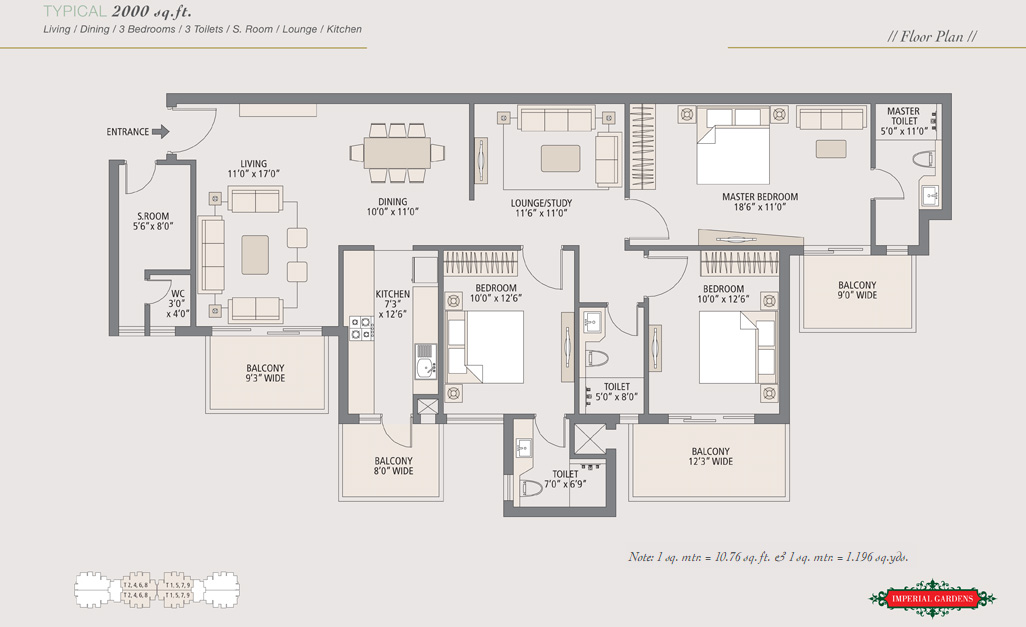This detailed illustration showcases a 2000-square-foot floor plan prominently labeled "Floor Plan" in the upper right corner. The layout features long gray lines that meticulously separate distinct areas within the space. 

Upon entering from the left side, where an entrance and directional arrow are indicated, one immediately steps into the living room, marked "Living 11x17." This area includes small square representations of furniture.

Adjacent to the living room is the dining area, depicted with a table and surrounding chairs symbolized by more squares. Moving further, the layout leads to the lounge/study area, progressing to the master bedroom on the right. Accompanying the master bedroom in the upper right corner is the "Master Toilet."

Below the master suite is a balcony, with another bedroom to the left and an additional bedroom continuing to the left. The kitchen, a long vertical rectangle, extends beneath these bedrooms. Another balcony is shown below the kitchen. To the right, a couple of inches away in a gray box, is another toilet, and nearby in a beige-colored box is the word "Balcony."

In the lower right corner, a red rectangle with white text provides additional details or notes, concluding the comprehensive depiction of the entire floor plan.